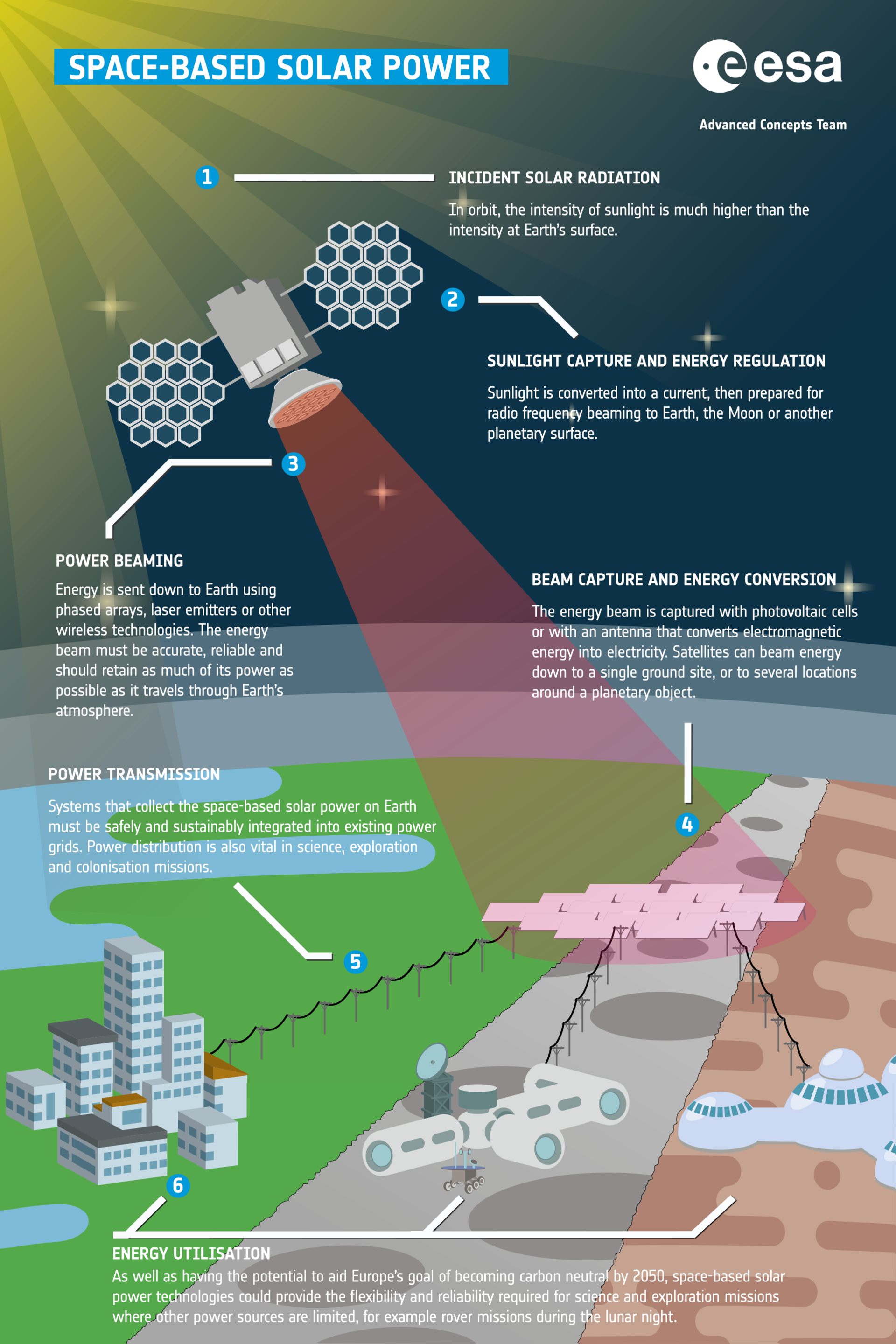This detailed, computerized drawing depicts a comprehensive overview of space-based solar power, labeled by the "Advanced Concepts Team" and prominently featuring the acronym "E-E-S-A". The large, attention-grabbing poster meticulously outlines six key steps in the process, each numbered within a blue circle and accompanied by an explanatory paragraph. 

1. **Incident Solar Radiation**: Highlights that the intensity of sunlight in orbit is significantly stronger than on Earth's surface.
2. **Sunlight Capture and Energy Regulation**: Describes the mechanisms for harnessing and managing solar energy.
3. **Power Beaming**: Illustrates the process of transmitting energy through beams.
4. **Beam Capture and Energy Conversion**: Details how these beams are collected and converted to usable energy.
5. **Power Transmission**: Explains the methods for transmitting the converted energy to its destination.
6. **Energy Utilization**: Concludes with the various applications of the transmitted energy on Earth.

The poster's layout includes cartoonish drawings of satellites beaming energy, buildings, roads, and other relevant images that make the complex process more accessible. The extensive use of colors and detailed graphics aims to captivate viewers' attention and educate them on the advanced concepts of space-based solar power.